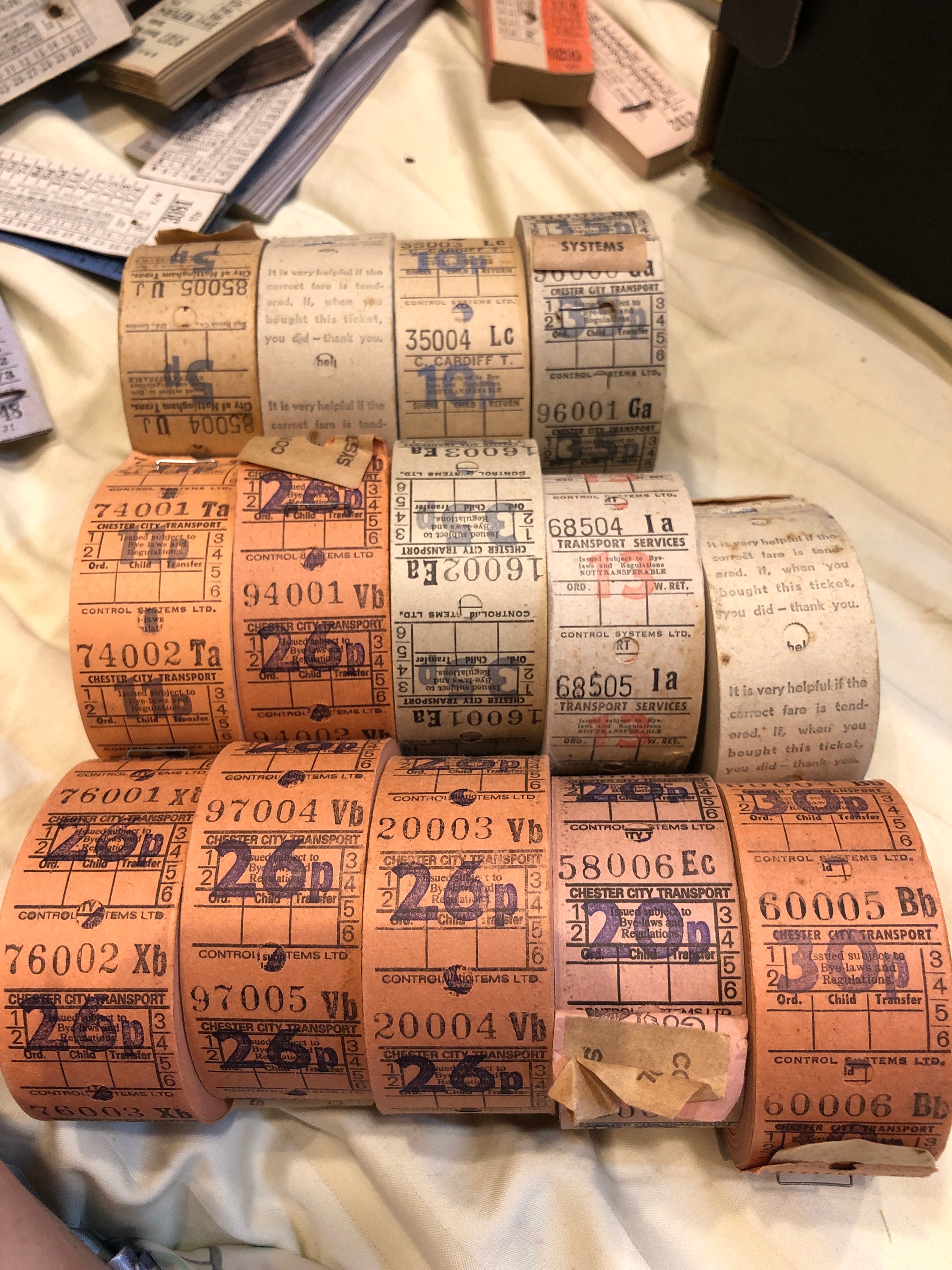The image depicts a collection of vintage transportation tickets, neatly arranged in three rows on a worn and stained white or cream-colored tablecloth. The bottom row consists of five rolls of tickets in various shades of pink, displaying prices 26P, 26P, 26P, 20P, and 30P. The middle row features four rolls with prices marked as 11P, 26P, 35P, and 13P, while the top row includes four smaller rolls labeled with 5P, 10P, and 35P. The tickets seem old, potentially from the early 20th century, and exhibit different stamps, with some reading "Chester City Transport" and "transport services." These rolls of tickets are visibly aged, suggesting a historical backdrop and possibly meant for old-timey transportation services. In the background, there are scattered ticket papers displaying unclear numbers.